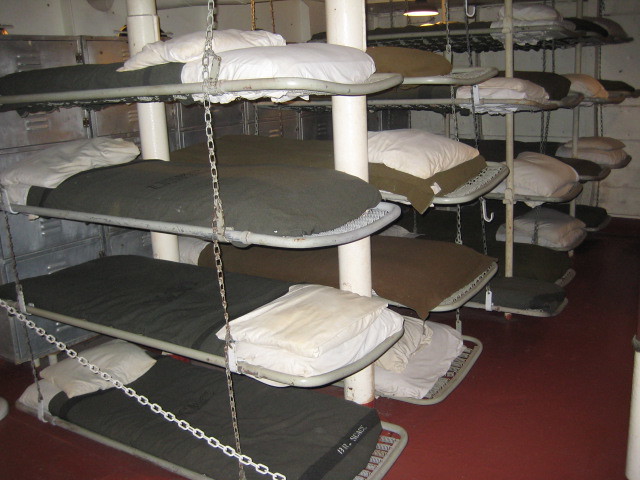The image depicts a tightly packed sleeping quarter that resembles a military or camp barracks. The space is filled with makeshift beds, each framed by thin, gray metal poles and stacked four to five levels high. The beds are supported by chains from the ceiling and consist of thin, paper-like mattresses with alternating thin and larger white pillows on each. Each mattress is adorned with either green or brown woolen coverings. The red floor contrasts with the white warehouse-like walls. On the side, vented foot lockers are visible. A white pole stands between these rows of stacked beds, suggesting an orderly but tightly confined setup possibly designed for accommodating between 20 to 30 individuals.